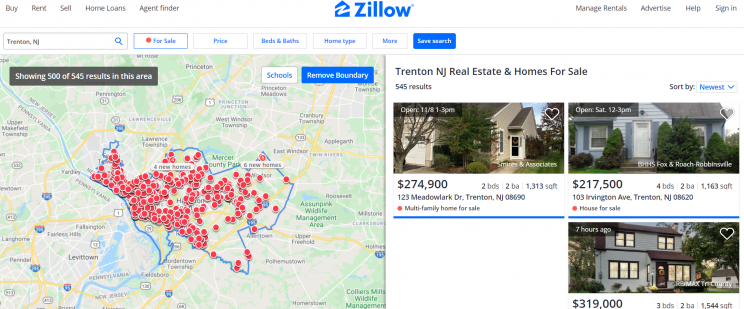This screenshot from the Zillow website showcases its interface for property searches. The Zillow logo, featuring a blue house with a white 'Z' inside and "Zillow" in blue text, is prominently displayed. Navigation options such as "Buy," "Rent," "Sell," "Home Loans," and "Agent Finder" are available for users.

The top search bar indicates a property search in Trenton, New Jersey, marked by a red dot next to the filter options which include: Price, Beds & Baths, Home Type, More, and Save Search. The search yields 500 out of 545 results in the specified area, as indicated by numerous red dots on the map.

On the right side, a section titled "Trenton, New Jersey Real Estate and Homes for Sale" displays three featured properties. The first listing, priced at $274,900, includes two bedrooms and approximately 1,313 square feet. The second property, listed at $217,500, is relatively new and features four bedrooms, two bathrooms, and 1,163 square feet. The third property, priced at $319,000, appears to be a modern or recently renovated home with three bedrooms and two bathrooms, encompassing 1,544 square feet. Each listing includes detailing such as addresses and is shown with an empty heart icon, indicating they have not yet been favorited.